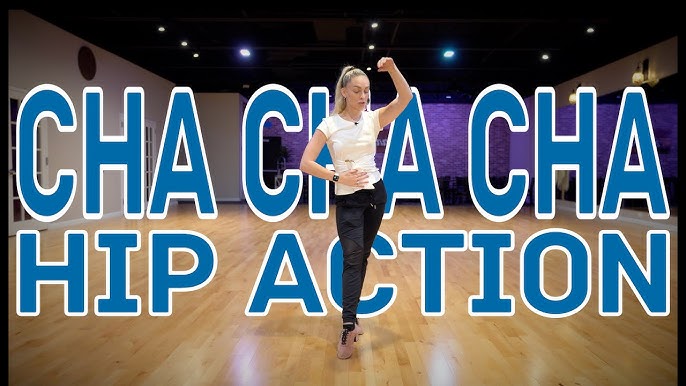The image showcases a woman with long blonde hair pulled back into a large ponytail, gracefully striking a dance pose on a highly polished wooden dance floor. She is front and center, appearing to be either in a dance class or performing for an instructional video, under soft purple lighting that accentuates her features against white walls. Behind her, large blue letters with white outlines spell out "CHA-CHA-CHA HIP ACTION," suggesting the focus on this particular dance move. The woman is dressed in a short-sleeved white t-shirt and loose black pants, paired with a stylish gold and black watch. In an elegant stance reminiscent of a ballerina, she has one hand raised above her head while the other rests on her stomach, positioning one leg forward and the other back, emphasizing her hip movement. Her downward gaze completes the poised and concentrated expression suited for a dance routine.